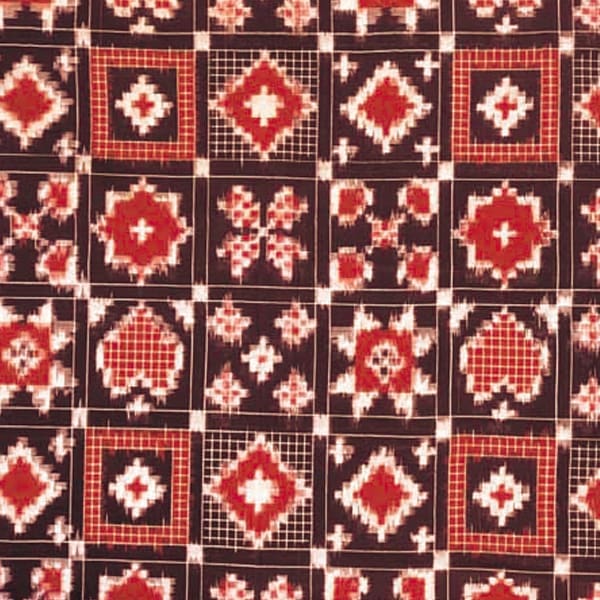This image is a slightly out-of-focus photograph of a quilt comprising 20 visible quilt squares arranged in a 5-by-4 grid, with partial quilt squares seen at the edges. The quilt squares are set against a brownish-black background and feature limited color variation, primarily brick red and white. The patterns within the squares include classic quilting shapes such as the Texas star, hearts, floral designs, and diamond shapes. Each square is clearly outlined by small white squares that demarcate their boundaries. The overall aesthetic of the quilt gives a sense of traditional, festive artistry, though it may not be considered one of the more visually appealing quilt designs.